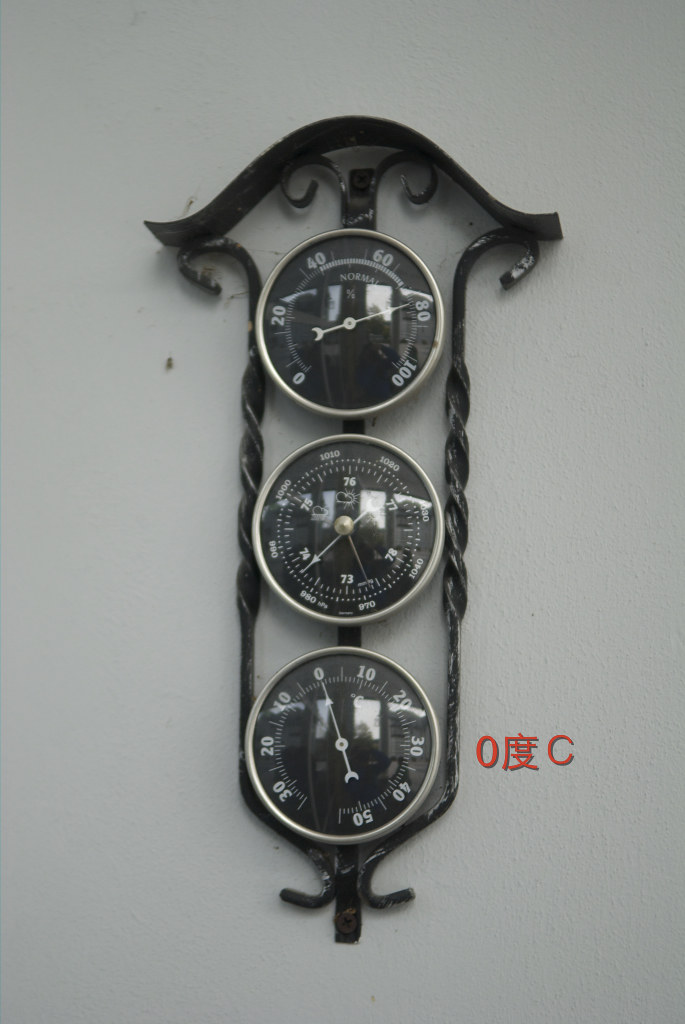This photograph showcases an intriguing and uniquely designed wall piece, resembling a clock at first glance but revealing itself to be more akin to automotive gauges. The gray wall backdrop suggests an indoor setting with minimal natural light, a notion supported by the overcast reflection visible on the surface of the wall piece.

The focal point is a vertically arranged trio of circular gauges, reminiscent of a stoplight. The surrounding frame of these gauges is a thin, black, loop-like design that loops back around itself, adding to the modern aesthetic.

The top gauge mimics a speedometer, with a golden needle pointing to the 80 mph mark. The middle and bottom gauges display different sets of numbers, though their exact functions are not immediately clear. The bottom gauge, in particular, features numbers ranging from 0 to 50, before counting back down to 30, 20, and 10, suggesting it might measure air compression or another pressure-related metric.

Overall, this intricate wall piece combines elements of automotive instrumentation with artistic design, resulting in a striking and thought-provoking art installation.